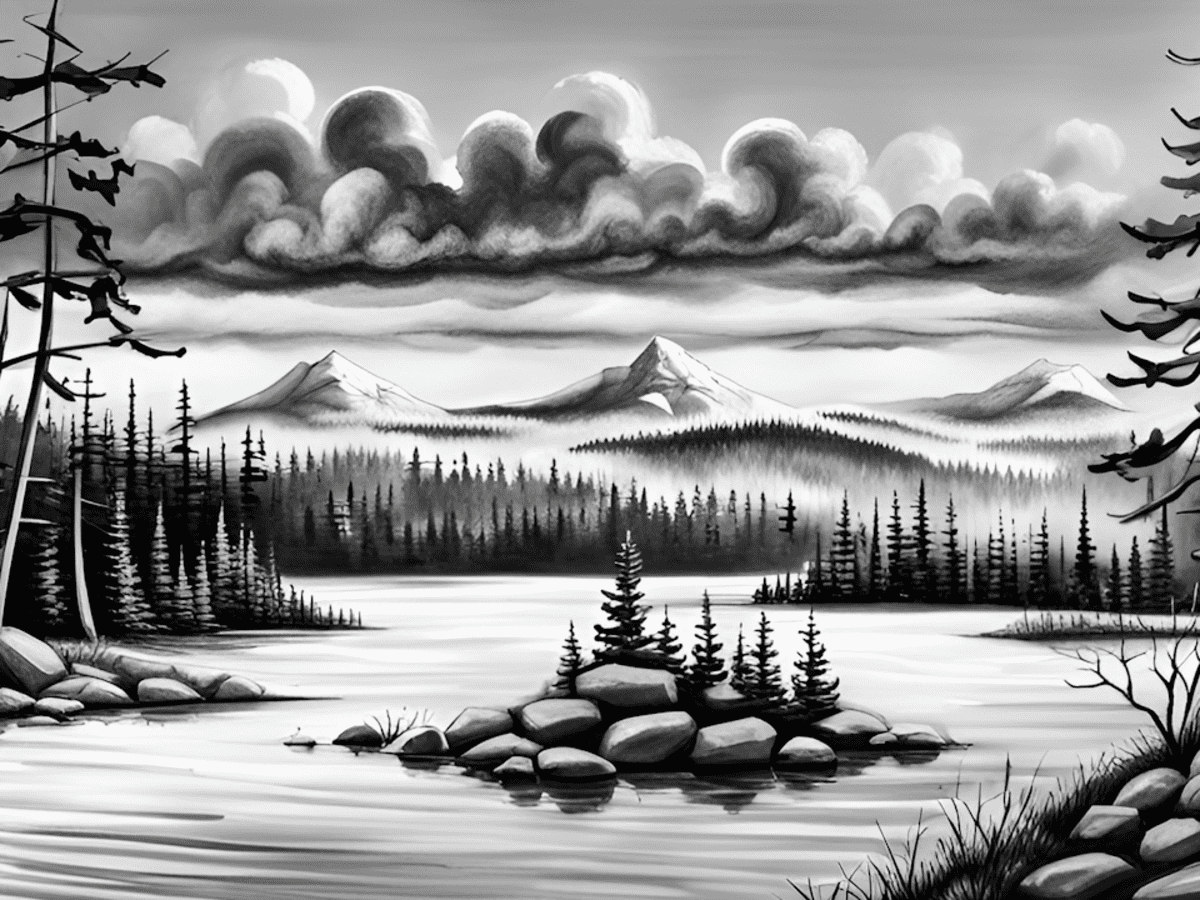This black-and-white image appears to be an intricate charcoal or pen sketch depicting a serene wilderness scene. At the center of the composition is a large, calm lake with only a few ripples, suggesting a peaceful ambiance. In the middle of this lake sits a small rocky island from which a cluster of small evergreen trees emerges, indicating that the water might not be too deep in certain areas. Surrounding the lake, the landscape is densely forested with evergreen trees continuing to the left, right, and all the way to the misty, distant horizon. Three towering snow-capped mountain peaks dominate the background, adding a majestic touch to the scene. Above, rolling dark clouds cover much of the sky, though the very top appears clearer. The image exudes a sense of tranquility and natural beauty, capturing both the ruggedness and calm of the wilderness.